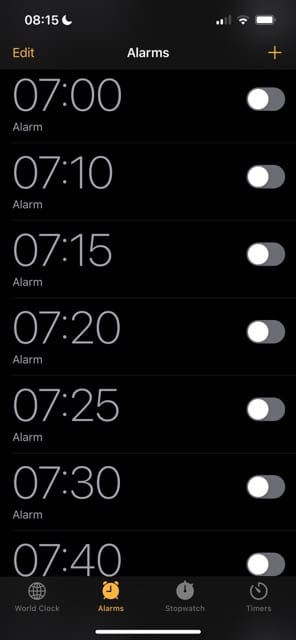This image is a screenshot of a phone or tablet displaying the alarms section of a clock app. At the very top of the screen, there is a dark gray status bar. On the left side of this bar, "0815" is displayed in white text with a half-moon icon next to it, indicating night mode or do not disturb status. On the right side, various icons show a two out of four bar network signal, a two out of three bar Wi-Fi signal, and a full battery indicator. 

Below the status bar, in the top left, the word "Edit" appears in gold color. Centered in the middle, the title "Alarms" is displayed, and on the far right, there is a plus symbol for adding a new alarm. 

The main section of the screen shows a list of set alarms, all written in light gray. The times are presented in large font, starting with "07:00." Each alarm time is accompanied by the label "alarm" in a smaller font directly underneath. The list includes alarm times of 07:00, 07:10, 07:15, 07:20, 07:25, 07:30, and 07:40. All alarms are currently switched off, suggesting the user may be in the process of selecting or modifying their alarms.

At the very bottom of the screen, another dark gray strip features four icons representing different sections of the clock app. From left to right: a globe icon labeled "World Clock," an alarm clock icon labeled "Alarms" in gold color (indicating the current section), a stopwatch icon labeled "Stopwatch" in gray, and a speedometer icon labeled "Timers."